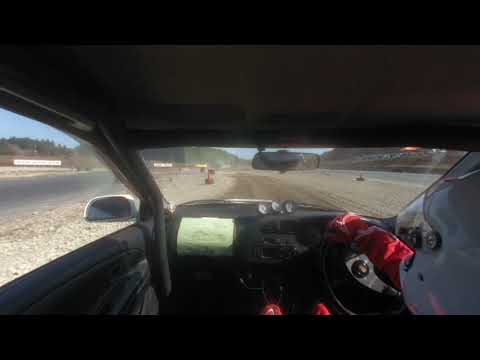This horizontal rectangular image captures the interior of a vehicle, likely a race car, from the perspective of someone sitting inside. The interior is predominantly black, with distinct features such as a screen on the left and a driver, wearing red gloves and a white helmet, gripping the steering wheel on the right. The steering wheel is on the right side, indicating it might be a European vehicle. Through the windshield, a dirt track extends ahead, flanked by trees and a building in the distance on the right side. On the left, visible through the side window and rearview mirror, is a mix of dirt terrain, trees, and possibly a farmhouse or barn under a blue sky. The image’s color palette includes black, brown, green, red, tan, gray, and white, with a notable red element inside the car near the bottom. There's also a hint of structures in the background, suggestive of bleacher stands and perhaps a train, reinforcing the outdoor setting of a race track.